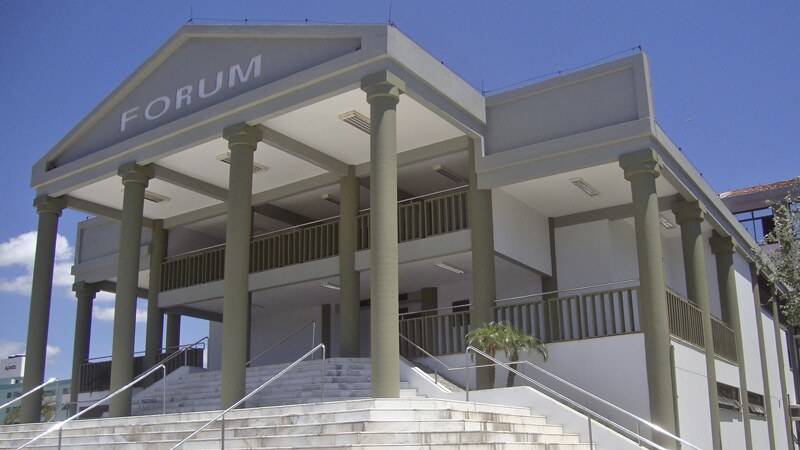The image features a grand building labeled "FORUM" in white letters prominently displayed above its entrance. The structure stands out with its imposing, tall pillars—four at the front—reaching a height of approximately 30 to 40 feet. These grayish pillars support a protruding promenade. The building's facade is painted in shades of olive green and deep gray, complemented by lighter gray trim, and features several balconies.

Leading up to the main entrance are multiple staircases with white steps, possibly marble or concrete, bordered by six to seven silver railings. The arrangement of these steps and railings creates a sense of grandeur and accessibility. To the side, there is a porch-like walking area, providing additional space outside the building.

The image is set against a clear, blue daytime sky with a few clouds visible on the left side, enhancing the urban environment. In the background, there are hints of other buildings and a tree to the right, adding depth to the scene. The overall composition highlights the architectural beauty and surroundings of the "FORUM" building.